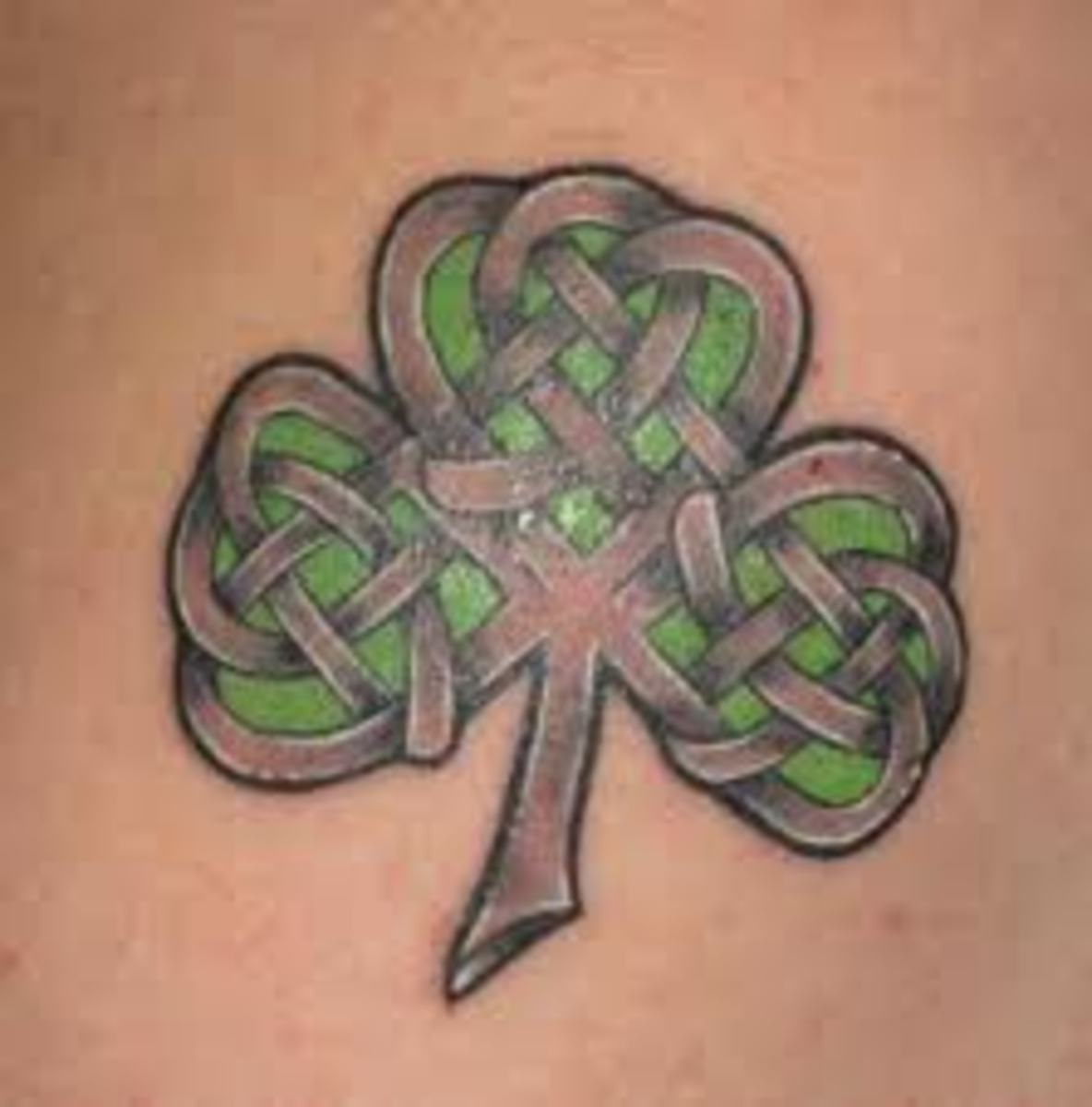This close-up photograph captures an intricate tattoo of a three-leaf shamrock on light, freckled skin, presumed to be of a Caucasian person. The shamrock, vertically oriented with its stem at the center bottom, features detailed Celtic knots that form a lattice pattern across its variegated greywashed leaves, creating a three-dimensional effect. Each petal of the shamrock intertwines with these knots, which are outlined in black and filled with different shades of gray, while the gaps reveal a light shamrock green. The tattoo stands out starkly against the skin, with no other elements or text present in the bronze-colored background.